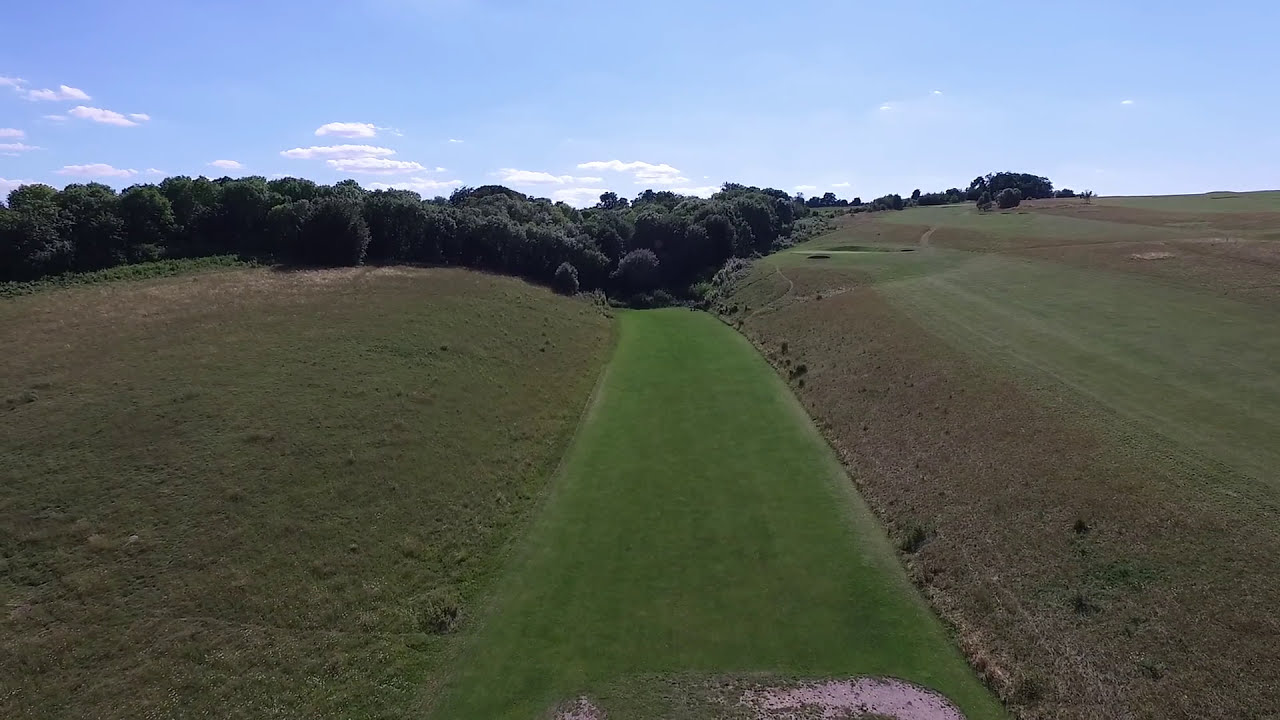The image depicts a vast, open rural area characterized by rolling hills and a serene, uninhabited landscape. The upper third of the photo showcases a mostly clear sky with a few scattered clouds, predominantly blue with hints of white. The background from center to left is dense with trees, continuing to the right but more sparsely. The central focus is a well-defined, evenly green path or valley strip, dissecting the scene. This path is flanked by fields of varying shades of green and brown, indicative of different crop areas or weedy, uncultivated land. Near the bottom of the path, there's a noticeable patch of gray dirt. The overall color palette blends green, brown, blue, white, and gray hues, with no buildings, people, or animals in sight. The photo, possibly captured from a drone or overhead perspective, emphasizes the natural beauty and tranquility of the rural countryside.